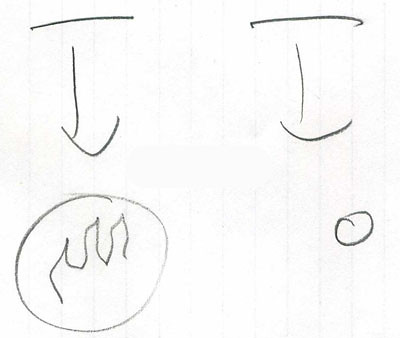The faint image displays a piece of lined paper with vertical gray lines, offering a distinct departure from the typical horizontal orientation. There are four pencil sketches on this paper. In the top left corner, there's a stylized letter "J," notable for its unconventional design where the upper curve does not connect with the vertical stroke. Adjacent to it, an eye is quickly sketched, with the upper and lower lids not meeting the central part, giving it a fragmented appearance. On the bottom half of the paper, a circle is filled with hand-drawn, flame-like patterns, featuring three prominent peaks. To the right of this, a small "O" or zero is depicted; the upper end of this character intriguingly extends inward. Despite the faintness of the grey lines on the paper, they provide a subtle guideline for the artwork.